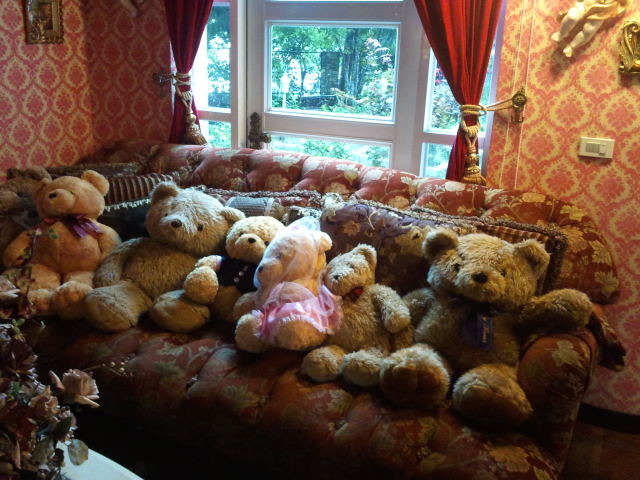This detailed photograph captures a cozy living room scene centered around a red and gold-patterned couch adorned with seven teddy bears of varying sizes and colors. The room features rich decor, with red wallpaper embellished with a subtle yellow tree-like pattern and matching red curtains tied off with golden ropes. The arrangement includes three large, darker-colored teddy bears and four smaller, lighter-colored ones, all neatly seated next to each other. In front of the couch, a table displays a lush bouquet, adding a touch of natural beauty to the scene. Behind the couch, a window framed in white with green foliage visible through the transparent glass further enhances the warm, homely atmosphere depicted in this front-facing photograph.